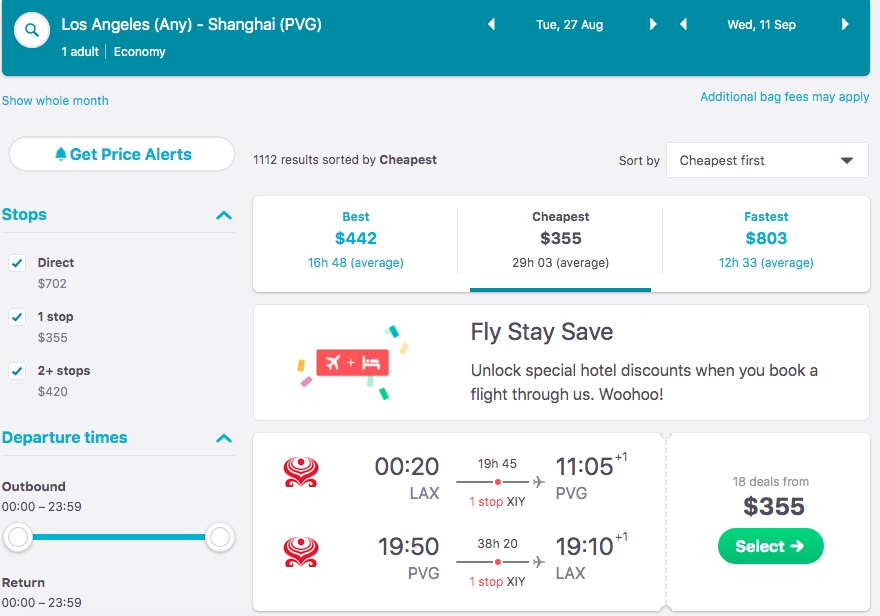Screenshot of an airline booking website displaying various flight options for one adult traveling from Los Angeles to Shanghai. The page showcases flights from multiple airlines, but the website itself remains unidentified. The available flights range in price, with the best rate being $442.00, the cheapest option at $355.00, and the fastest route costing $803.00. On the left side of the screen, there are filters to narrow down the search results, including options for direct flights, one-stop flights, and two-stop flights, as well as departure time preferences.